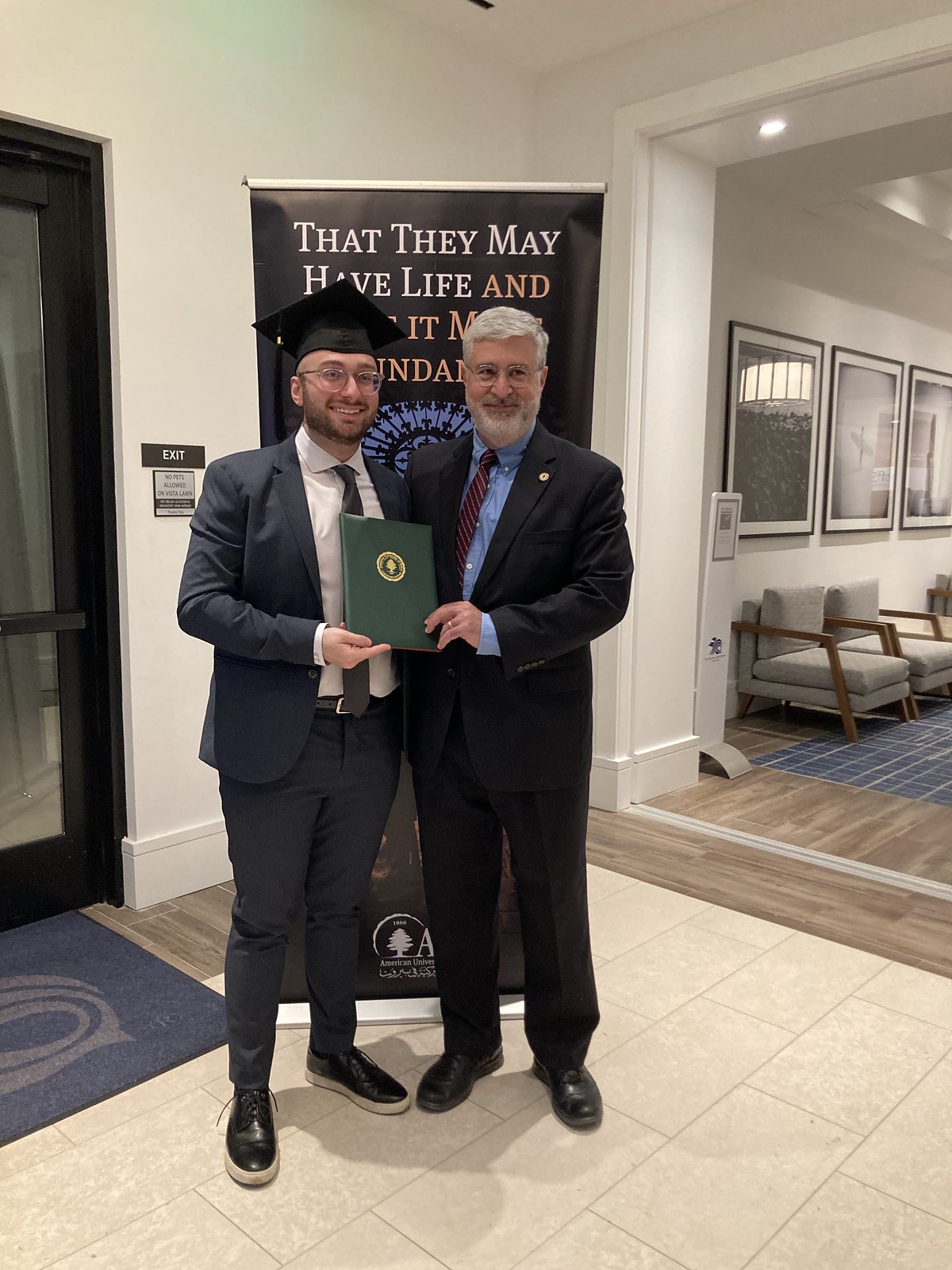In an educational setting, likely a college, a young man with glasses and a short beard stands proudly next to an older man with light gray hair. The younger man, dressed in a sharp blue suit, white dress shirt, black tie, and black shoes, is celebrating his graduation, signified by his graduation cap and the green leather diploma cover with a gold emblem that both men hold together. The older man, also in glasses, wears a black suit, blue dress shirt, and a maroon striped tie. Behind them, a partially visible banner reads "that they may have life," believed to be part of a Biblical verse, with "American University" and additional text that appears to be in Arabic, at the bottom. To the left, an exit sign reads "No Pets Allowed on Vista Lawn." To the right, a room with cushioned, low-seating chairs can be seen, along with framed artwork on the wall. The atmosphere is bright with light streaming in, highlighting the celebratory and academic ambiance of the scene.